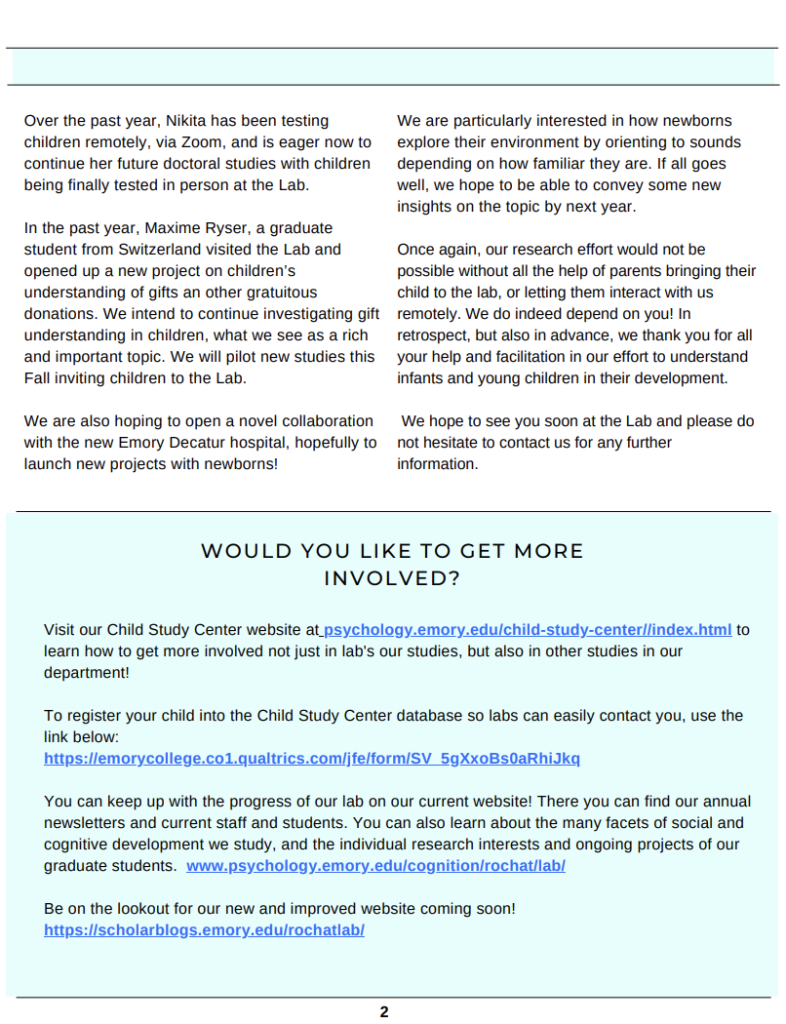Here is a cleaned-up and detailed descriptive caption for the image:

---

The image showcases a digital text document, which appears to be part of a blog or an article. The document begins with a light blue banner across the top, although it lacks a title or any identifying text to indicate its origin, potentially from a website. Below the banner, several paragraphs are presented, detailing research activities and future plans involving child studies.

The text highlights the work of Nikita, who has been testing children remotely via Zoom over the past year while looking forward to resuming in-person testing for her doctoral studies at a lab. It mentions Maxime Reiser, a graduate student from Switzerland, who visited the lab to initiate a new project on children's understanding of gifts and donations. The document outlines the intention to continue exploring this topic and pilot new studies in the fall, inviting children to the lab. Furthermore, there is an aspiration to collaborate with Emery de Kouder Hospital to launch new research projects involving newborns, particularly focusing on how newborns orient to sounds based on familiarity with their environment.

The document expresses the hope of sharing new insights by the following year and details additional ongoing and future research efforts at the lab. At the bottom of the document, there is a prominent blue section offering ways to get more involved, with various links for registering children, viewing progress, and details about an upcoming website improvement. Each of these links is underlined and clickable. Notably, a number "2" appears at the very end of the document, possibly indicating pagination.

---